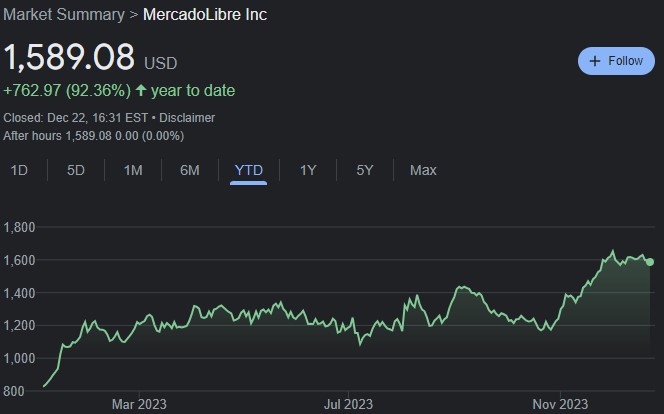The image is a large, cropped screenshot of the Market Summary tab for Mercado Libre Inc. within a dark-themed interface. Dominating the left side of the image are the figures "1589.08" displayed in large, white numerals, indicating the current stock price. Adjacent to this, in smaller grey text, is the currency notation "USD." Beneath this, the growth information is prominently featured with the text "+762.97 (92.36% up year to date)" in green, highlighting a substantial increase. 

Further details include the closing time note: "Closed December 22nd at 1631 Eastern," which appears just above an after-hours price information section. Beneath these details is a line chart that visualizes the stock's performance. 

At the top, there are eight selectable categories displayed: "1 Day," "5 Days," "1 Month," "6 Months," "Year to Date," "1 Year," "5 Years," and "Max." The "Year to Date" option is highlighted in blue, indicating the current selection. The line graph below reflects the stock's performance over the specified year-to-date period.